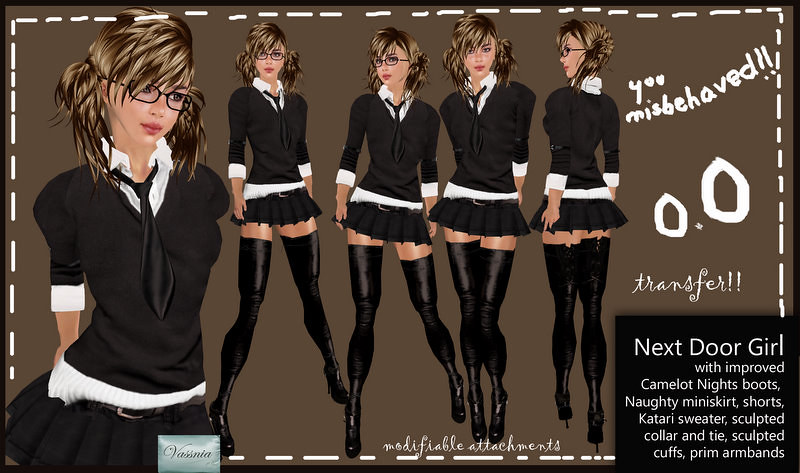The image is an advertisement or a business card, possibly related to an adult show or Halloween costume. It features a computer-generated, animated character of a girl dressed in a short skirt and a Qatari sweater with a black tie. The character also wears high socks over her legs, Camelot night boots, and sports knotty miniskirts, shorts, and sculpted cuffs with prim arm bands. The text on the image reads "You misbehaved" and includes phrases like "next door girl" and "improvised Camelot night boots, knotty miniskirt, shorts, Qatari sweater." The card itself is designed in shades of brown, white, and black.